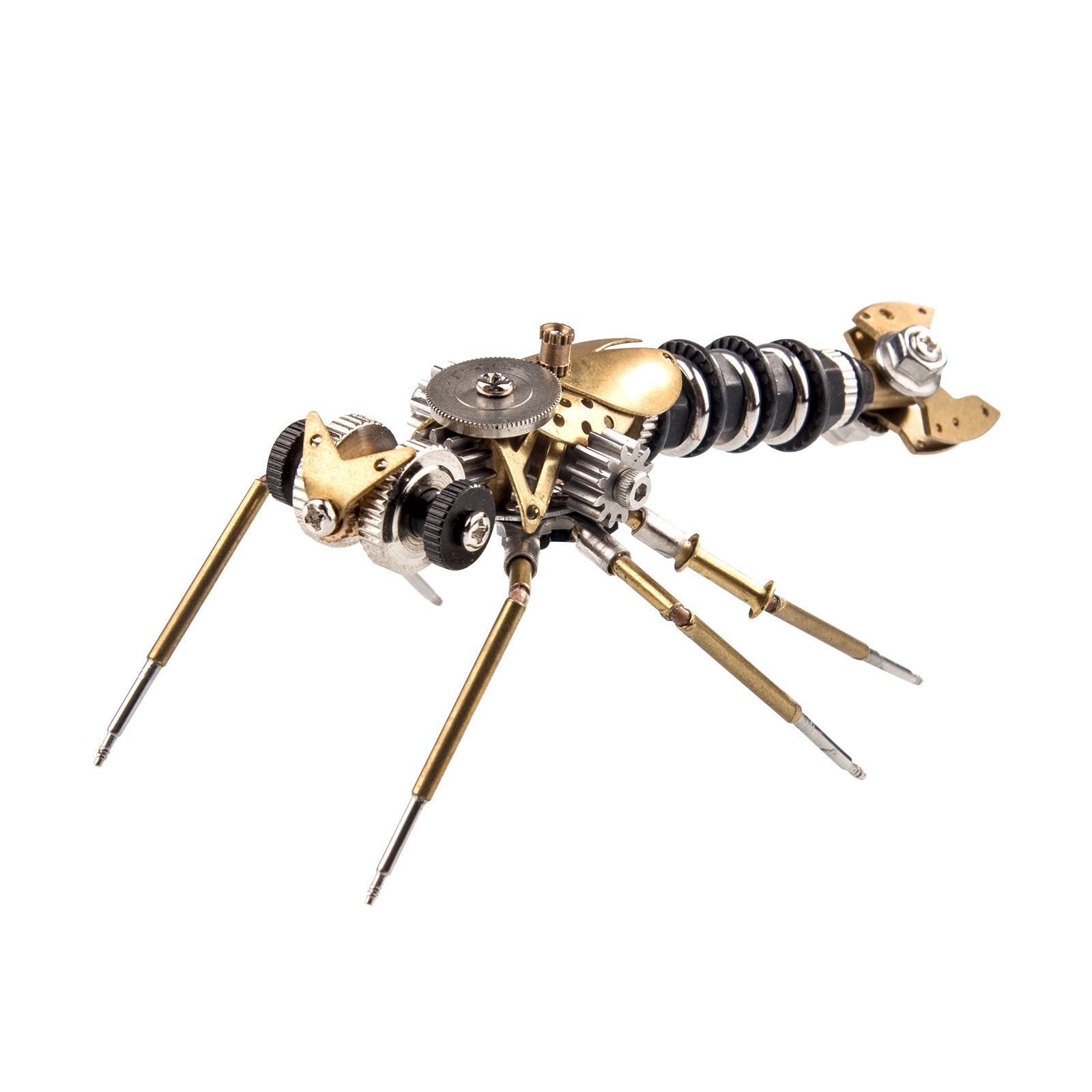The image depicts a detailed and intricate metallic construct resembling a robotic insect or scorpion. The body of the insect is composed of an array of gears, nuts, bolts, and various metallic segments in copper, gold, and silver hues. The head features two prominent round gears, with a silver gear situated towards the top of its back. The abdomen showcases three black rubber-like sections that mimic an insect's segmented body. Extending from the body are four leg-like appendages that are crafted from gold and silver metals, ending in pointed tips that resemble claws. Additional black wheels and discs are attached to the underside, further emphasizing its mechanical aesthetic. The tail section is adorned with copper elements, giving it a distinctive scorpion-like appearance. This complex assembly of metallic parts, gears, and mechanical components suggests it is an artistic representation rather than a functional device.